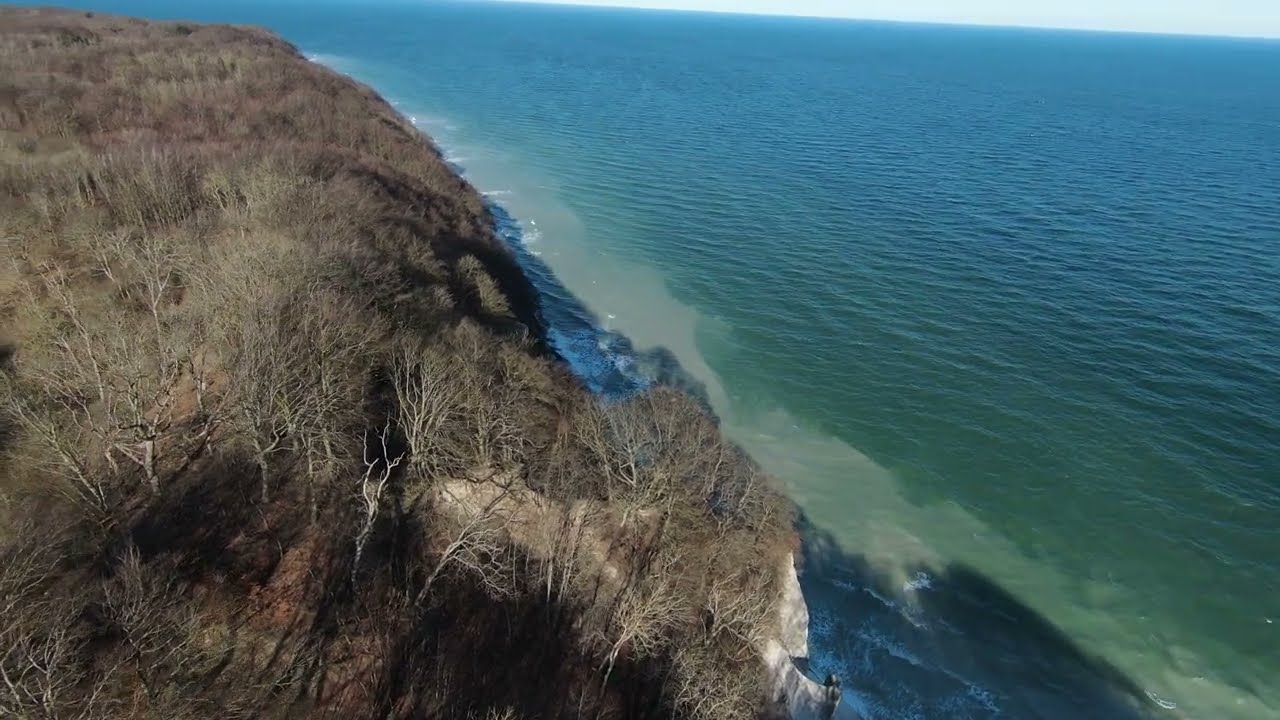This detailed photograph captures a stunning view of a coastal cliffside. To the left of the image, a steep hill rises, covered with dry, brown grass and leafless deciduous trees, indicative of winter. The ground is similarly brown and drab, devoid of greenery, with the occasional large rock, including a notable large flat boulder and a round rock hanging off the cliff. The sea, stretching out to the right, showcases a gradient of colors from deep teal green in the distance to a milky, lighter green close to the shore, with waves breaking at the base of the cliff. The horizon extends far into the distance, underscoring the vastness of the ocean. Towards the central lower portion of the image, one person can be faintly seen, adding a sense of scale to the landscape.